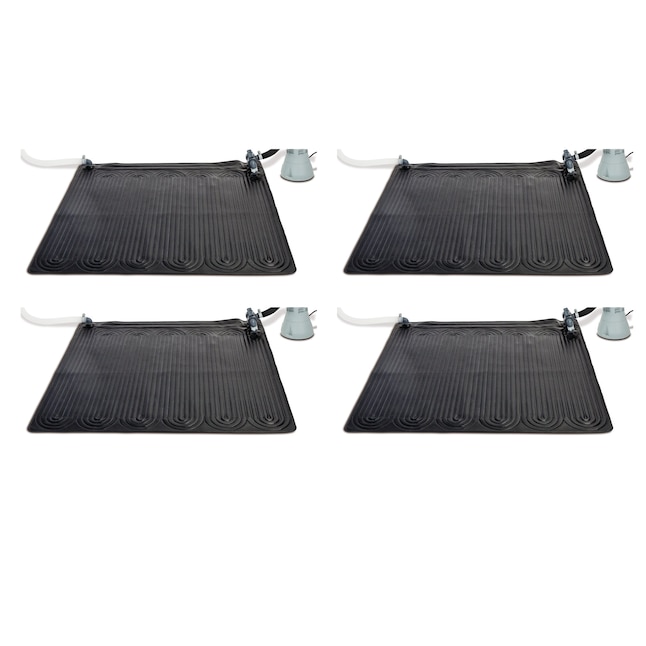The image displays four almost identical black rubber mats, each featuring a looping texture that forms elongated oval patterns. Positioned in a 2x2 grid, the mats have a white, clear, or black tube at the top left corner, which spirals vertically, traversing the mat's surface in a sinuous manner. Upon reaching the right edge, the tube exits the mat and appears to connect to a green beaker or pale blue container, suggesting a liquid flow system. This intricate tubing within the mats likely facilitates a cooling or heating mechanism, as the liquid seems to be pumped across the entire mat surface before being collected and channeled out. Despite the repetition, no clear distinctions are noticeable between the four mats, emphasizing their uniformity. The exact function remains ambiguous, with no additional textual or visual clues provided.